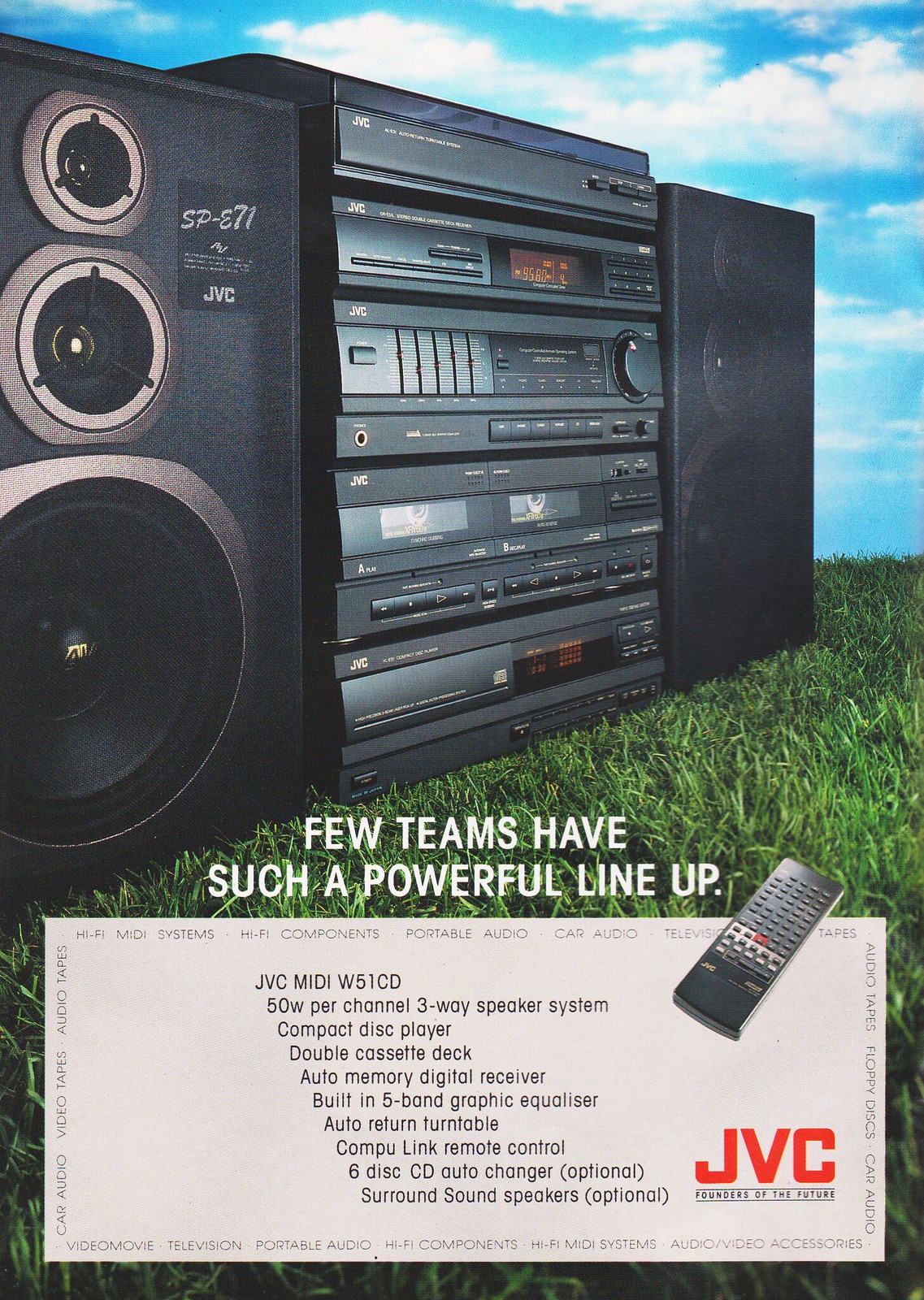The image is a screenshot of a vintage advertisement, likely from the 1980s, featuring a sophisticated stereo system by JVC. The advertisement showcases a detailed picture of the system set in a flat, grassy field under a vast blue sky with light clouds. The camera captures the scene at the same elevation as the stereo system, angled for a clear view of its components. The stereo system is a tower setup consisting of several key elements: 

- A CD player situated at the bottom,
- A dual cassette deck player above the CD player,
- A power amplifier equipped with a five-band equalizer positioned above the cassette deck,
- A digital radio receiver at the next level,
- And at the very top, a record player with an auto-return feature.

Flanking the central tower on either side are two large black speakers, each with three separate speaker sizes for optimal sound quality. The text at the bottom of the advertisement lists the impressive features of the system, highlighting the JVC MIDI W5-1CD model, which boasts a 50-watt per channel three-way speaker system, a compact disc player with a six-disc auto changer, a double cassette deck, an auto memory digital receiver, a built-in five-band equalizer, and the CompuLink remote control. The tagline reads, "Few teams have such a powerful lineup."